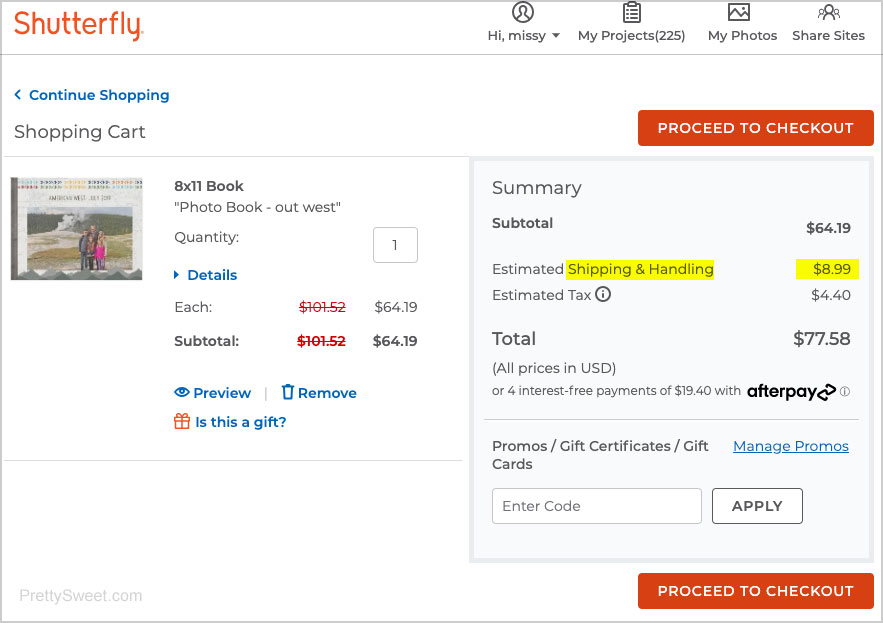The image depicts a Shutterfly web page. In the upper left-hand corner, the Shutterfly logo is prominently displayed in red. Adjacent to the logo are various interactive tabs; the first tab reads "Hi, Missy," indicating the user is logged into her account. Under "My Projects," it shows that Missy has 225 active projects.

Below this section is an icon of a shopping cart. Inside the cart is an 8x11 photo book titled "Out West," featuring a cover image of two people standing amidst a hilly landscape. The book is listed with a quantity of one and has a discounted price of $64.19, marked down from an original price of $191.52. 

Highlighted in red at the upper right corner is a "Proceed to Checkout" button. To the right of the image, there is a summary of Missy's order total, with the shipping and handling fee highlighted in yellow at $8.99, bringing the overall total to $77.58.